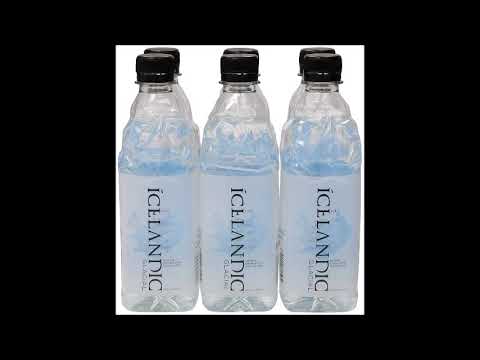The image displays six photorealistic, clear bottles of Icelandic brand water, each with a black cap. These bottles are organized in two rows of three, with the back row's caps just visible from a slightly elevated angle. The word "Icelandic" is printed in black vertical font along the side of the bottles, and additional, smaller text is discernible though not legible. The bottles are rectangular, tapering smoothly towards the cap. They feature a clear plastic wrap predominantly white with an icy blue section in front, surrounding the main body. These bottles are set against a pure white background occupying a white square, itself inset within a slightly larger black rectangle that is wider than it is tall.